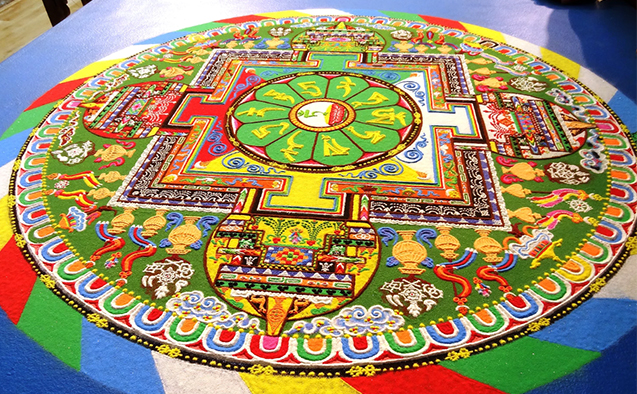The image depicts a large, round, possibly embroidered piece that resembles a blend of a rug and a game board, adorned with vibrant and eye-catching colors. The piece boasts an intricate blue border that encloses several nested circles, each featuring a kaleidoscope of colors including red, green, blue, yellow, white, and more. The outermost circle displays a series of wedges repeating in white, yellow, red, green, and blue. Within this, a black line interwoven with gold threads forms a ring of small bow-like patterns, and inward of this are segments that resemble horseshoes or mini rainbows adding to its oriental charm. A central square encompasses yet another circle, adorned with myriad designs rich in green, yellow, purples, and lime hues. The entire composition is reminiscent of traditional Asian design elements, potentially evoking Japanese or Chinese cultural influences, and although it could be a game board, its artistic embroidery suggests it may also serve as a decorative piece. The overall effect is a mesmerizing display of brilliant, bright colors and elaborate details sure to captivate any viewer.